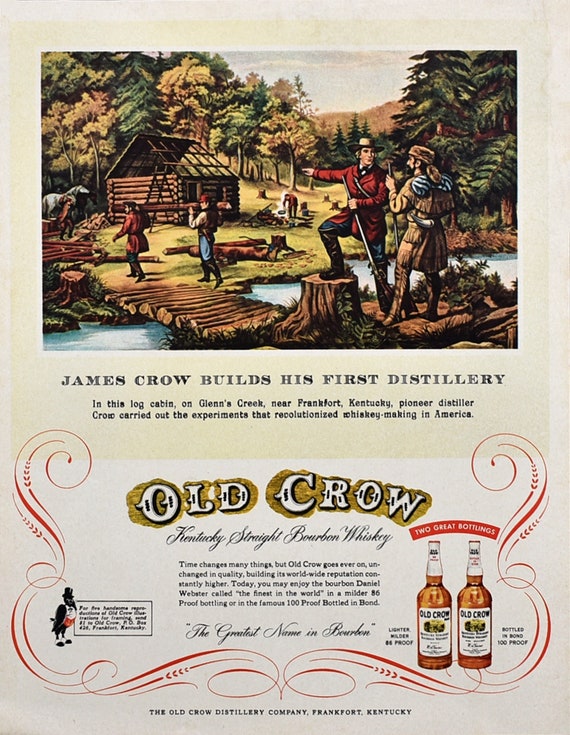The image is a scan of an old magazine advertisement featuring an intricate artwork at the top. The colored drawing showcases a historical outdoor scene where a man in a red jacket and a fur hat is standing on a tree stump, pointing towards a log cabin being built by several men around it. This pioneer setting includes a creek, a log bridge, and a forest in the background. The text below the artwork states, "James Crowe builds his first distillery." It explains that in this log cabin on Glens Creek near Frankfort, Kentucky, pioneer distiller James Crowe conducted experiments that revolutionized whiskey making in America. Further down, there's a logo for "Old Crow" with the accompanying text, "Kentucky Straight Bourbon Whiskey." Two bottles of the whiskey are shown in the bottom right corner beneath the phrase "two great bottlings." The ad continues to highlight the enduring quality and storied history of Old Crow, quoting it as "the greatest name in bourbon" and concluding with, "The Old Crow Distillery Company, Frankfort, Kentucky."